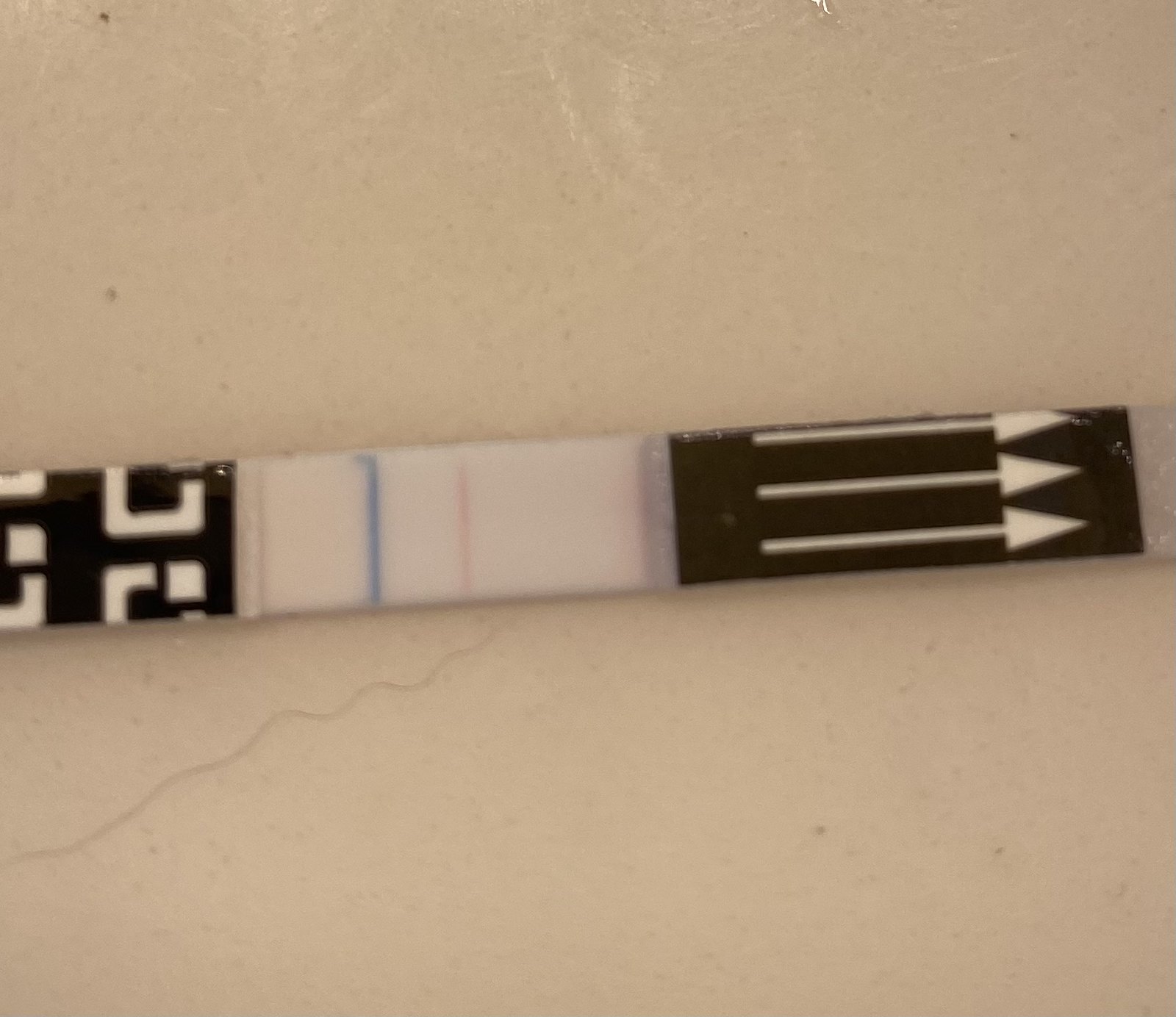In this image, we see a white countertop with a pattern of fine, squiggly lines resembling either marble veining or fallen strands of straight hair. The countertop is otherwise clean except for a few visible stains and marks that suggest it could use a wipe-down. Prominently displayed on the counter is a Covid test, characterized by a long rectangular shape. On the left end of the test, there is a black section with indiscernible white lettering. Along the test strip, a blue and a red line are visible, indicating a positive result. Further to the right, the test strip has black sections with white arrows pointing towards an unseen section of the test, presumably directing where the sample would need to be inserted. The composition of the image hints at a casual and spontaneously captured moment, possibly showcasing a significant and concerning result within a domestic setting.